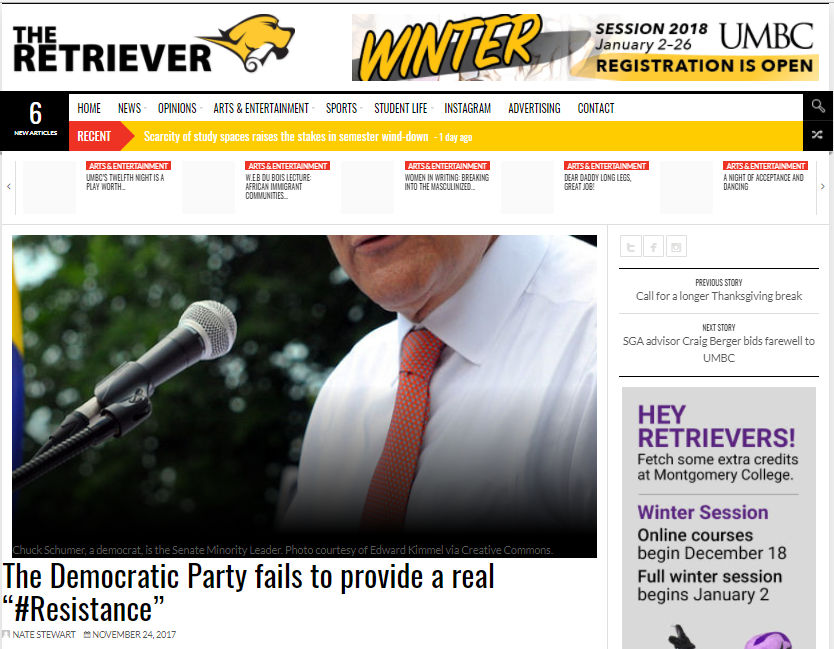The image is a rectangular screenshot of a webpage, identified as the front page of "The Retriever," a publication from UMBC. It predominantly features a white background with various colored sections for organizational clarity. In the top left corner, bold black text reads "The Retriever," accompanied by a cartoon of a yellow dog holding a rolled-up newspaper in its mouth. Next to this, the word "Winter" is displayed in gold-yellow with a black outline.

To the top right, details are provided in black text: "Session 2018, January 2 till 26," with "Registration is open" on a yellow background beneath it, and "UMBC" appearing prominently. Below this header, there is a thin black line demarcating the next section, which includes navigational links: Home, News, Opinions, Arts & Entertainment, Sports, Student Life, Instagram, Advertising, and Contact.

A central feature is a large photograph showing only the lower half of a Caucasian man's face, focusing on his lips and chin. He wears a white dress shirt and a red tie, speaking into a microphone. Below this photo is the headline: "The Democratic Party Fails to Provide a Real #Resistance," attributed to Nate Stewart, dated November 24, 2017.

The webpage includes various secondary articles and sections. A red arrow-shaped banner with white text indicating "Recent" complements another segment, "Scarcity of Study Spaces Raises the Stakes in Semester Wind Down," highlighted in white text on a yellow background. An extensive content bar displays article headlines across subjects, notably with red banners labeled "Arts and Entertainment," detailing diverse campus cultural events.

Adjacent to the main photo, additional navigation aids and article previews are present, providing a comprehensive snapshot of campus news and features. A promotional section at the bottom right corner, featuring a gray background and purple text, invites readers to "Fetch some extra credits at Montgomery College," emphasizing winter session registration starting December 18, and full session beginning January 2.